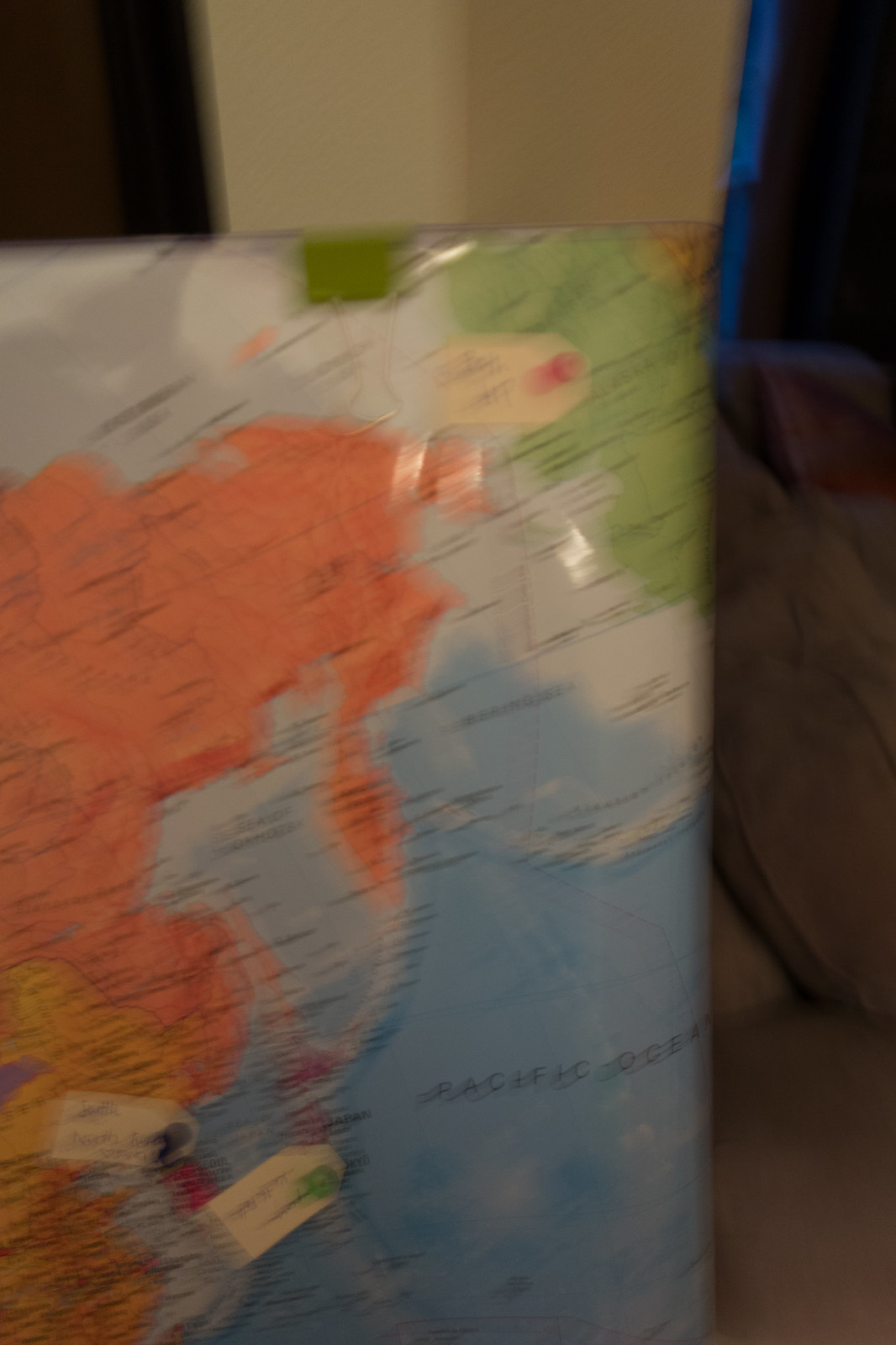This is a blurry portrait photograph likely caused by camera movement, depicting a shiny, laminated or plastic world map positioned in front of a living room couch. The main focus of the image is the Pacific Ocean, which is visibly located in the bottom right corner of the map. The map appears slightly rolled up, obscuring some parts on the right side. Various landmasses are visible, including Eastern Russia, Eastern China, Japan, and Korea, with Russia depicted in orange, China in yellow, and parts of North America, specifically Canada, in green. Several labels, thumbtacks, and tags are scattered around Eastern China and adjacent regions. There is also a green metal binder clip attached to the top of the map near Alaska or Canada, along with another label that is not readable due to the blurriness of the photograph. Additionally, many cities are listed in black text across the map, with noticeable reflections visible on its surface.